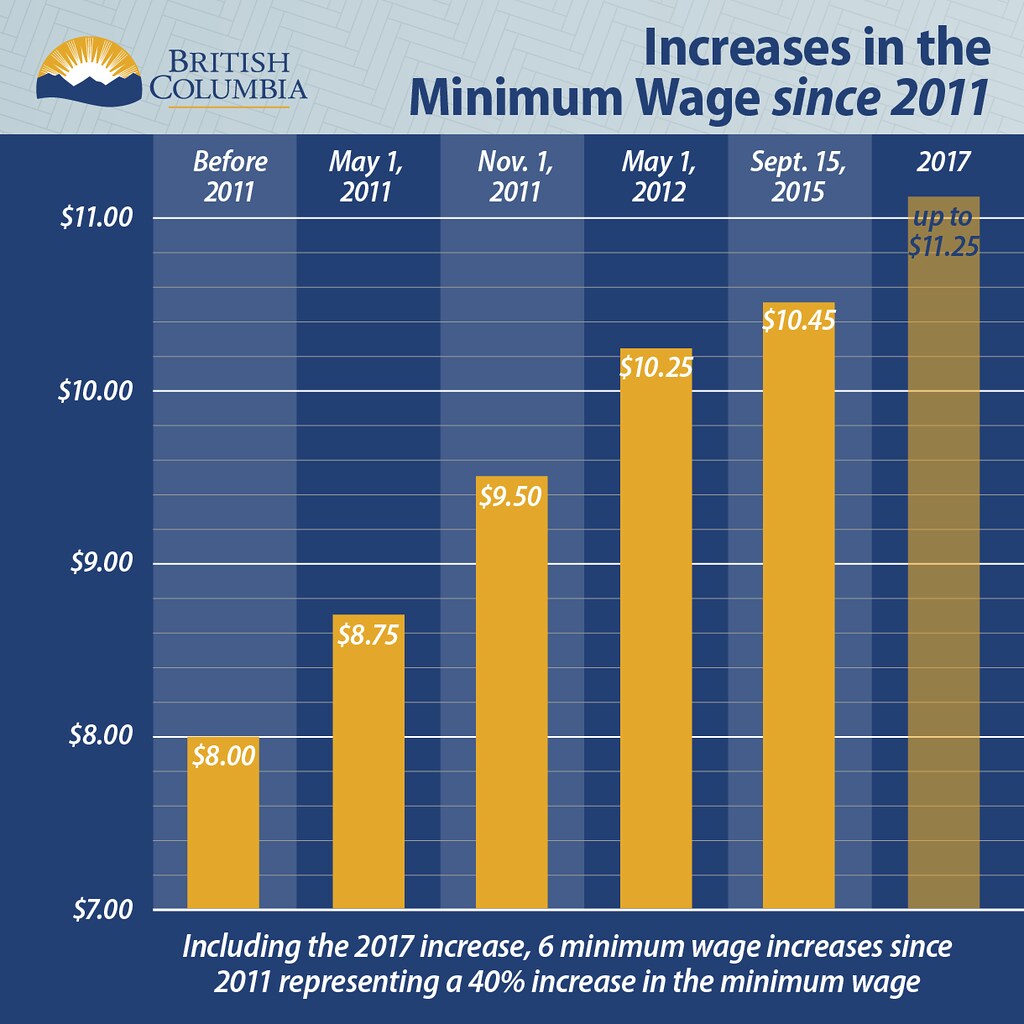The image is a detailed bar graph displaying the increase in the minimum wage in British Columbia since 2011. At the top left corner, there is a logo featuring a sun with rays above mountains, labeled "British Columbia." The chart is predominantly dark blue with yellow-orange bars indicating wage amounts. The y-axis ranges from $7 to $11 in $1 increments, while the x-axis marks key dates: "before 2011," "May 1st, 2011," "November 1st, 2011," "May 1st, 2012," "September 15, 2015," and "2017." The graph shows the minimum wage rising from $8 before 2011 to $11.25 in 2017. At the bottom, the text in white states, "Including the 2017 increase, six minimum wage increases since 2011, representing a 40% increase in the minimum wage." The chart's overall layout is accentuated by a light blue border at the top, contributing to its visual clarity.